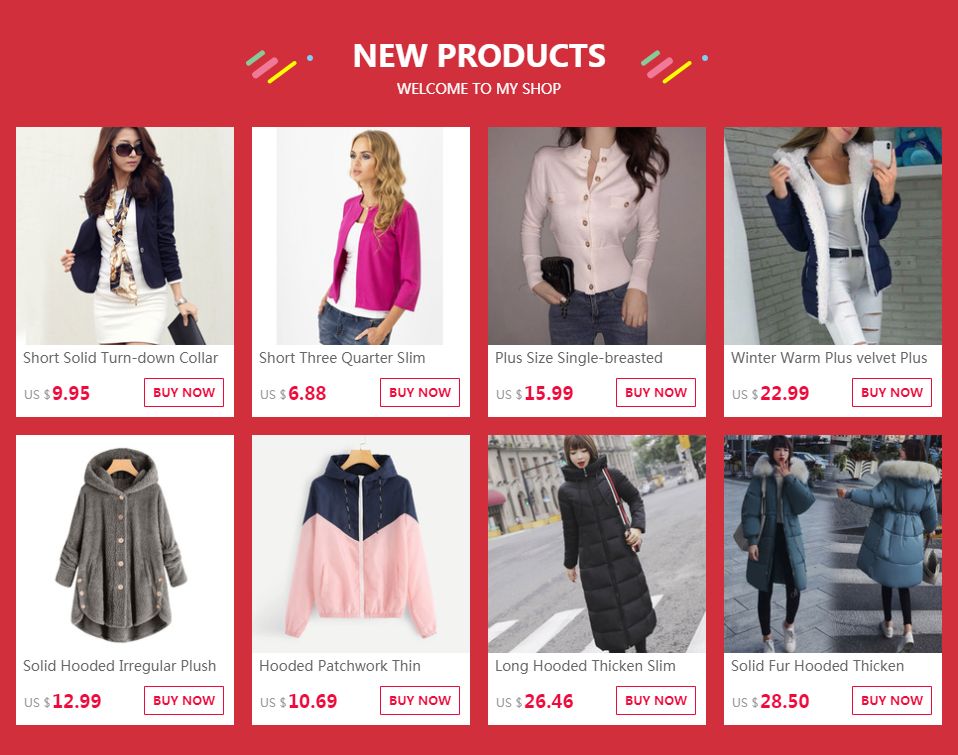The image features a collection of women's clothing items against a plain red background, which prominently displays the text "New Products" at the top. Below this header, it welcomes visitors with the phrase "Welcome to my shop." The image displays several clothing items, including six that are modeled by individuals. The models consist predominantly of Asian women, with a couple of Caucasian women also featured. Notably, two items, identified as a solid hooded irregular plush sweater and a hooded patchwork thin sweater, appear without models and are presented against a white background.

The models are photographed in diverse settings; some are situated outdoors in what appears to be an urban environment, while others are positioned against an unembellished white indoor background. The prices of the items are marked in US dollars, with the highest-priced item listed at $28.50. The most affordable item is a short, three-quarter sleeve slim sweater priced at $6.88. Each product listing is accompanied by a "Buy Now" button. The simplistic and somewhat bare design of the site suggests that it may still be under development.